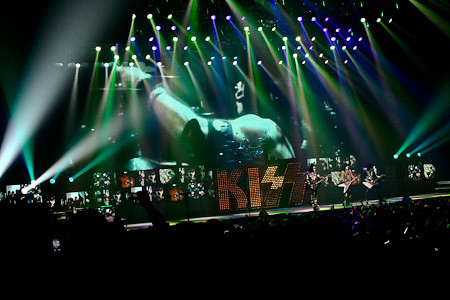This photograph captures the vibrant energy of a KISS concert. The stage is illuminated with a dynamic array of green, blue, pink, and purple lights shooting down from the ceiling, spreading across the top part of the image. Dominating the background is a large monitor screen displaying a close-up of one of the band members, who is turned to the left with his arm extended upwards. Flanking the screen is the iconic light-up KISS sign, although partially obscured, and multiple smaller monitors seem to be scattered throughout the stage backdrop. On the right side of the stage, three band members are seen playing their guitars. The bottom half of the image is notably dark, overshadowing the crowd, amplifying the dramatic lighting and stage effects. This intense scene perfectly encapsulates the electrifying atmosphere of a KISS concert.